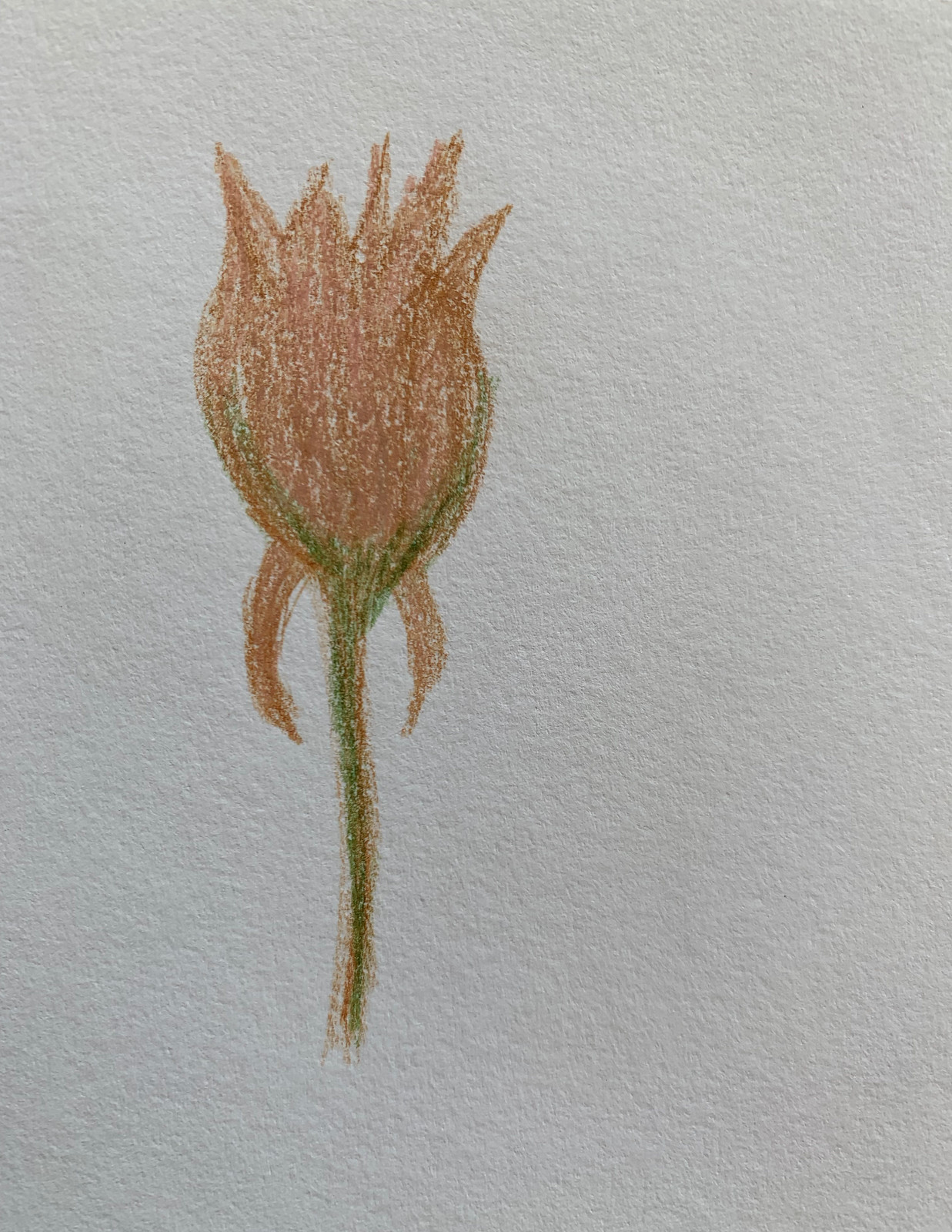A simple yet captivating image showcases a hand-drawn flower gracing the left-hand side of a textured white surface, possibly a piece of paper with a unique finish that almost resembles a wall. The flower illustration employs a subtle palette of green and reddish-brown hues. The dark green stem, tinged with touches of the reddish-brown shade, twists into a U-shape at its base, lending an organic fluidity to the design. The flower itself, rendered in the same light reddish-brown pigment, features five upward points and two downward extending segments, closely resembling the elegant form of a tulip.